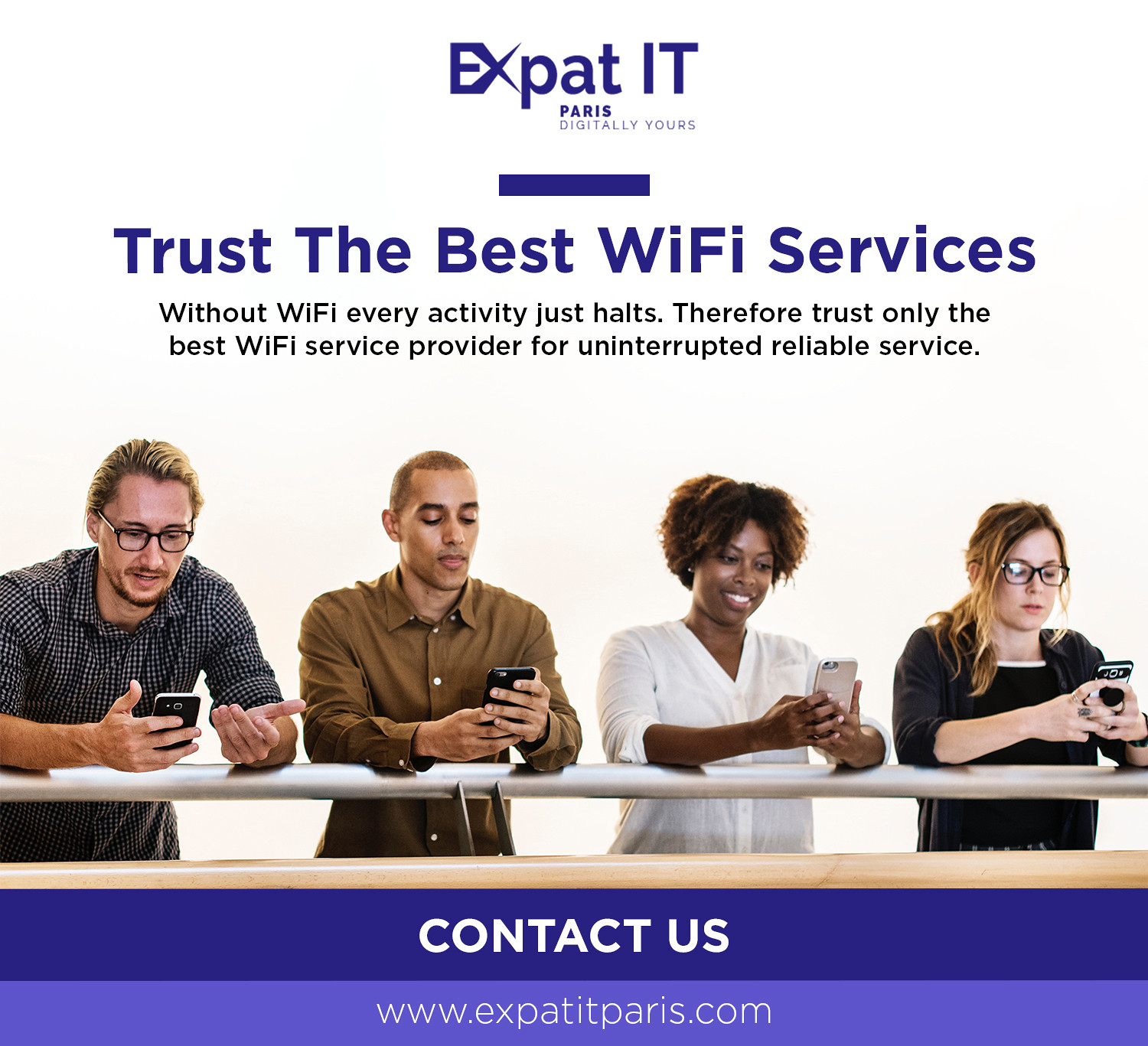This professional advertisement features a large, square layout with a clear and concise message. At the top, in prominent blue letters on a white background, the text reads "XPAT IT Paris, Digitally Yours." A line separates this header from the main content. Below, in bold blue letters, it states, "Trust the best Wi-Fi services." This is followed by a key message in black: "Without Wi-Fi, every activity just halts. Therefore, trust only the best Wi-Fi service provider for uninterrupted, reliable service."

In the central image, four people lean against a metal railing, each engrossed in their cell phones. On the left, a white man with dark hair, blonde highlights, dark-framed glasses, a beard, and a mustache wears a plaid blue shirt. He appears annoyed or confused, gesturing with one hand. Next to him, a black man with dark hair and eyebrows in a brown shirt holds his phone with both hands and licks his lips.

To the right, a smiling black woman with dark hair and a white blouse holds a silver phone, possibly taking a selfie. Finally, a young white woman with long brownish-blonde hair, glasses, and a pop socket on her phone wears dark clothing and is absorbed in her screen. At the bottom, a dark blue banner with white text reads "Contact Us," followed by a lighter blue banner stating "www.expatitparis.com." This ad targets expatriates in Paris seeking dependable Wi-Fi services.